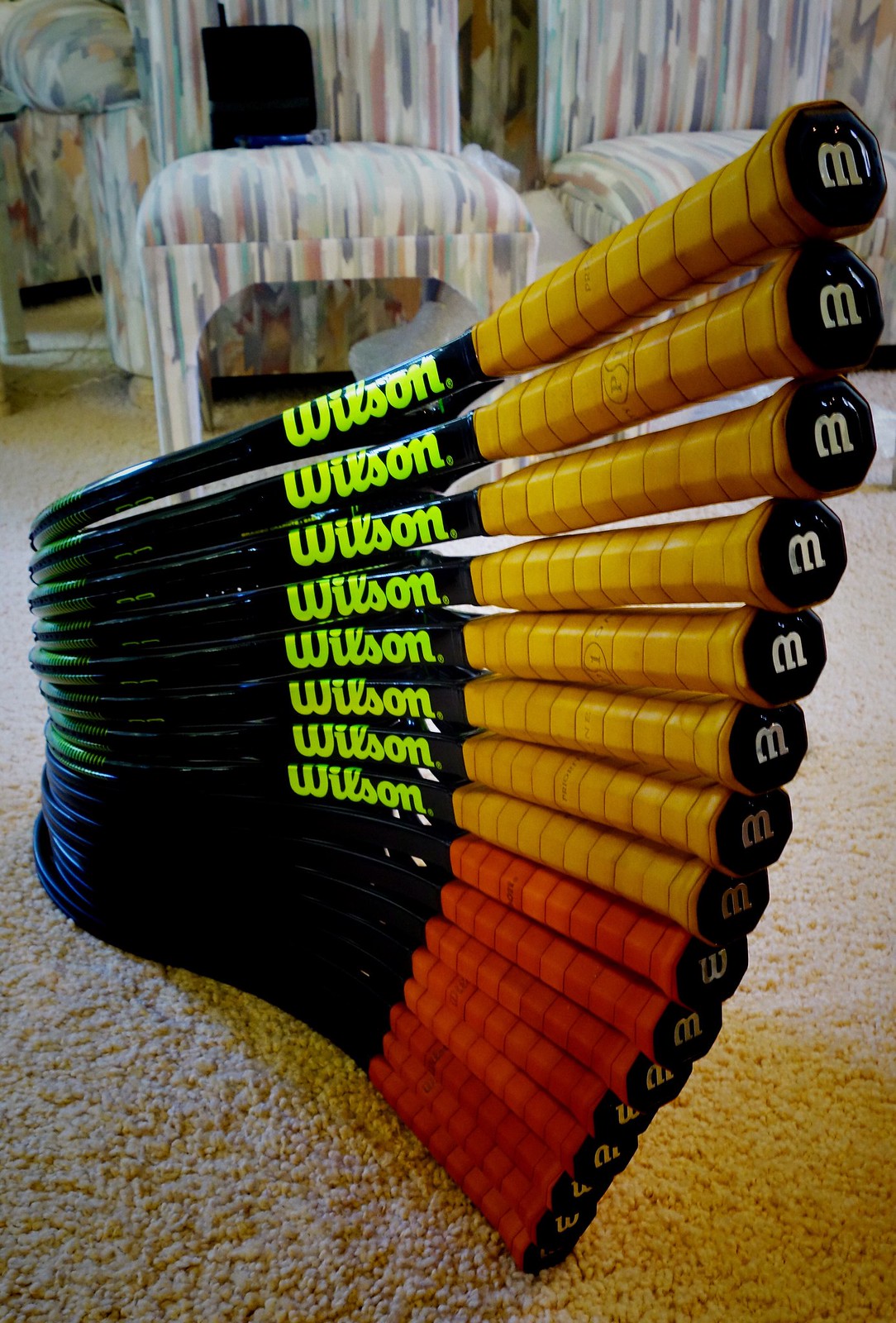This detailed image showcases a neat arrangement of Wilson tennis rackets, stacked in a symmetrical, fan-like display on a beige carpet in the center of a living room. The rackets have red and yellow handles, with a bright yellow Wilson logo visible on the yellow-handled ones. About sixteen rackets, with black frames, are arranged with their tops pointing towards the left center of the image. The bottom of each handle is marked with a 'W'. In the soft-focused background, there are colorful chairs adorned with stripes in blue, pink, white, and gray. A shadow of the rackets is cast on the carpet, enhancing the structured yet curvaceous display.